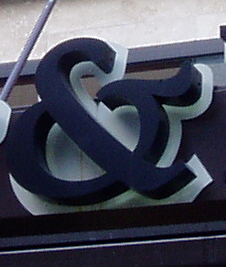This image captures a close-up view of a store sign prominently featuring the "@" symbol, stylized to resemble the letter "E" in black lettering. The bottom edge of the distinctive symbol rests atop a black section of the sign. The background reveals the upper portion of a building, characterized by its beige and white coloration, suggestive of a brick construction. Additionally, to the left of the "@" symbol, a long gray pole emerges from another part of the sign, adding to the structural detail present in the scene.